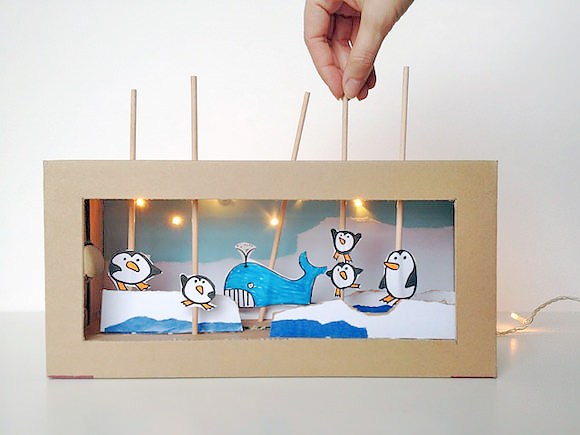This is a meticulously detailed colour photograph, likely created by AI, depicting a miniature puppet theatre. The backdrop divides into a dual-toned grey: a slightly lighter grey at the top transitioning to a darker grey at the bottom. Central to the composition is a human hand, visible at the upper centre, grasping a long, thin stick. This stick penetrates a frame and orchestrates a quirky, penguin-like cartoon character at the end. 

Surrounding the central character, a collection of shorter, rounder penguin figures congregates, each affixed to its own stick. Amidst these animated creatures, a blue whale emerges in the middle, complete with a water spout feature. Each puppet is designed for manipulation via attached sticks, suggesting this setup is intended for creative storytelling or playmaking.

The rectangular frame, within which this whimsical scene unfolds, hosts small lights at the top. It showcases a grey and blue backdrop adorned with elements of snow and water, enhancing the thematic setting. Notably, a cord extends from the right side of the frame, providing power to the illuminating lights. The overall scene portrays an innovative mini theatre, inviting users to craft their own narratives by maneuvering the characters with sticks from above.